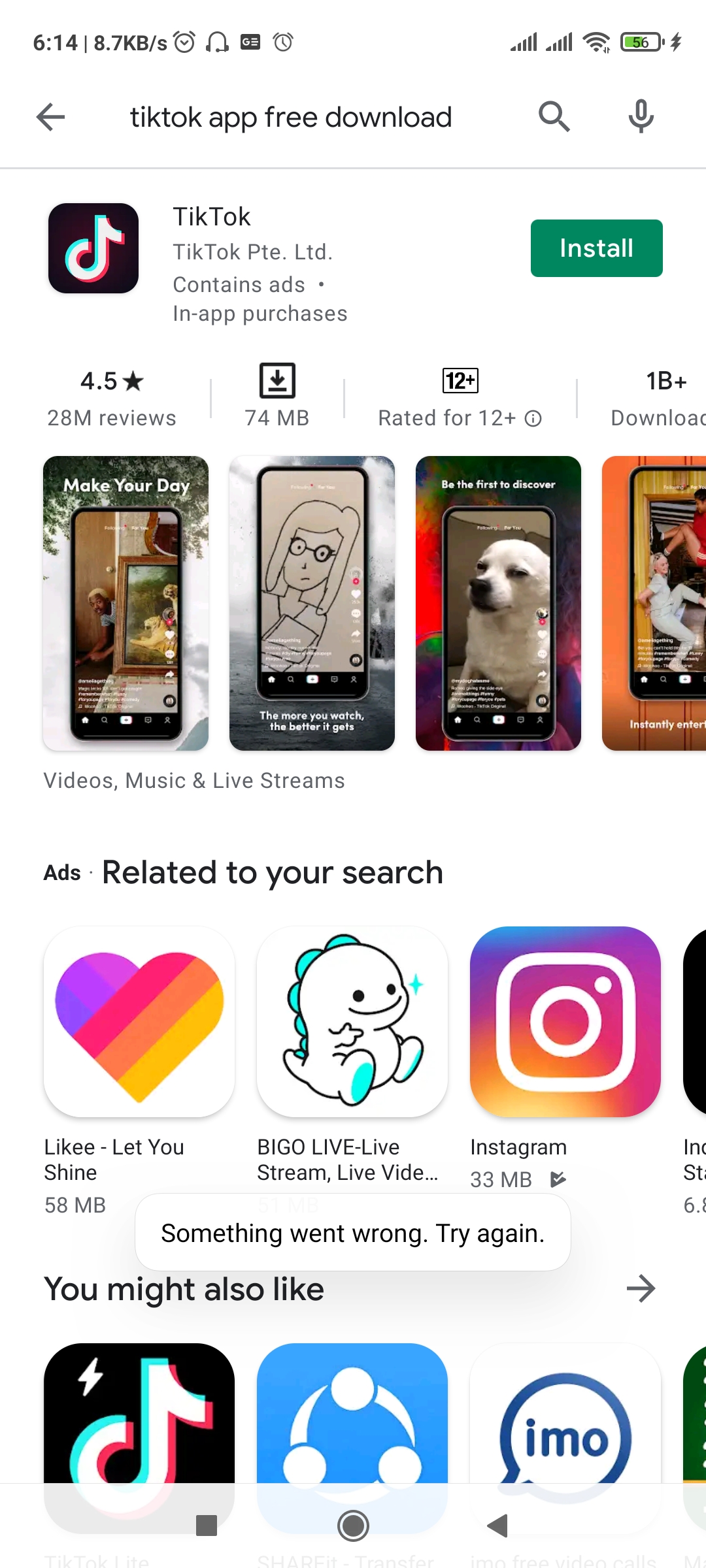This is a vertically oriented screenshot, likely captured from a smartphone. The background appears plain white, probably due to the default computer display.

**Top of the Screen:**
- The status bar indicates the time as 6:14. 
- There's a file size indicator showing 8.7 KB.
- Several icons are present including a clock, headphones, and an alarm icon.
- On the right, two signal strength bars, a Wi-Fi symbol, and a battery icon displaying a green charging indicator are visible.

**Main Content:**
- Below the status bar is a back arrow pointing left, adjacent to the text "TikTok - Free Download" in black.
- To the far right, there are a magnifying glass and a microphone icon.

**TikTok App Details:**
- The recognizable TikTok icon is accompanied by the app name "TikTok".
- It is noted that the app "Contains ads · In-app purchases".
- A green "Install" button is situated on the right side.
- The app has a rating of 4.5 stars based on 28 million reviews and requires 74 MB to download.
- The app is rated for ages 12+ and boasts over 1 billion downloads.
- Descriptive text highlights features such as "Beauty videos, music, and live streams."

**Additional Information:**
- There's a section with advertisements related to the user's search.
- An error message in a white box reads, "Something went wrong. Try again."
- At the bottom, there's a "You might also like" section with additional app suggestions, accompanied by icons including a square record button and a left-pointing triangle.